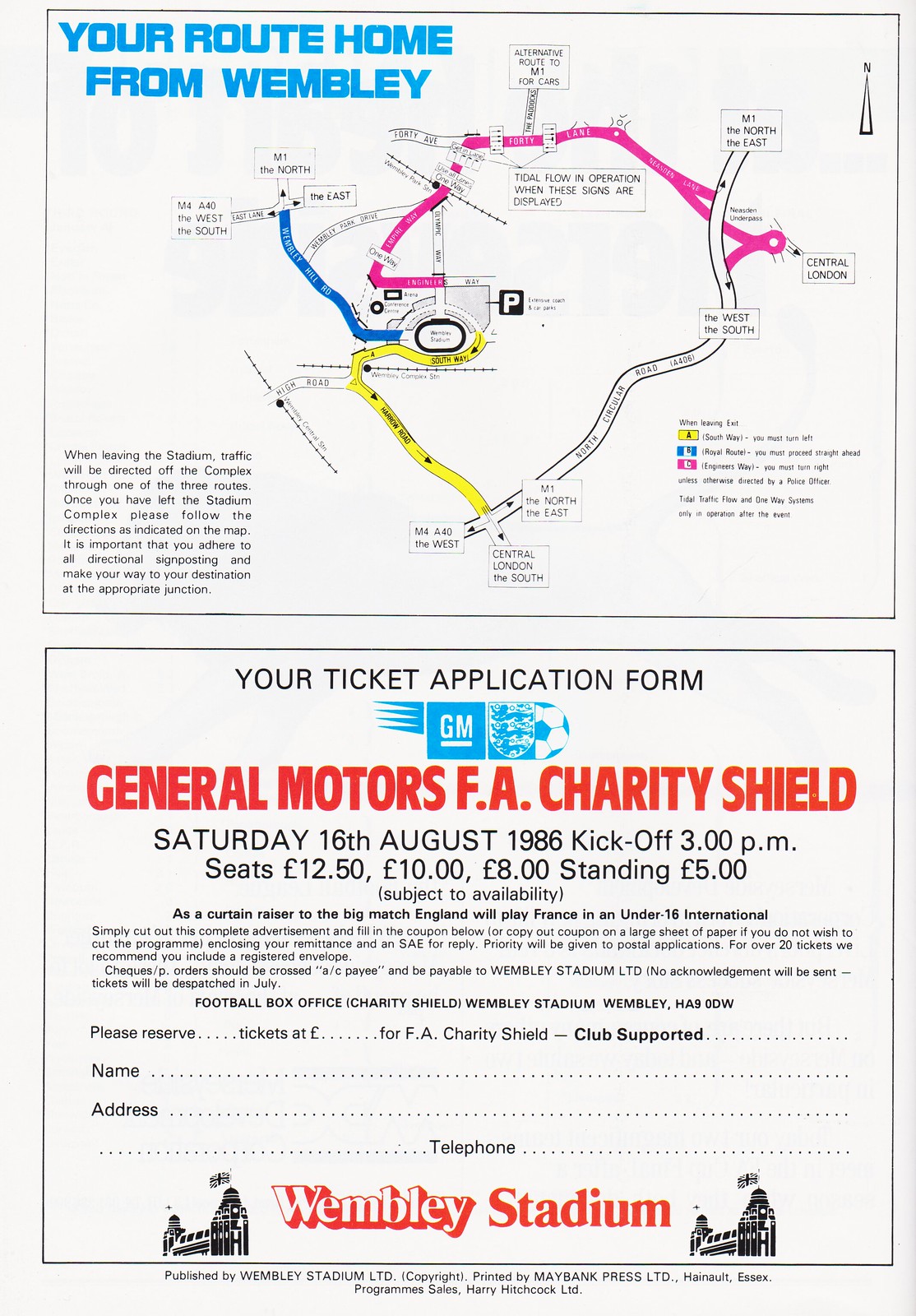The image is a detailed application form for the General Motors F.A. Charity Shield dated August 16, 1986. The upper half of the image features a heading in blue, all capital letters in the top left corner, reading "YOUR ROUTE HOME FROM WEMBLEY." Below the heading, there's a map outlining three color-coded routes: yellow in the lower left, blue in the middle, and pink along the top and right upper portion. A white road is also visible. Additionally, a block of text occupies the lower left corner, explaining directions to follow upon leaving the stadium. A key for the map is situated in the lower right corner of this section. 

In the bottom half of the image, centered text in a black border box prominently states in red capital letters, "GENERAL MOTORS F.A. CHARITY SHIELD." Below this, in black font, it details the event: "Saturday, 16 August 1986. Kickoff, 3 p.m. Seats, £10, £8 and standing, £5." Further down, a red-font paragraph describes logistical details, culminating with "Wembley Stadium" accented in red font and flanked by clip art of the stadium's spires. The application form structure is well-organized, with spaces for personal information, ensuring clarity for applicants. The entire page is visually mapped out with a variety of colors including white, pink, black, yellow, blue, and red, making it both informative and easy to navigate.